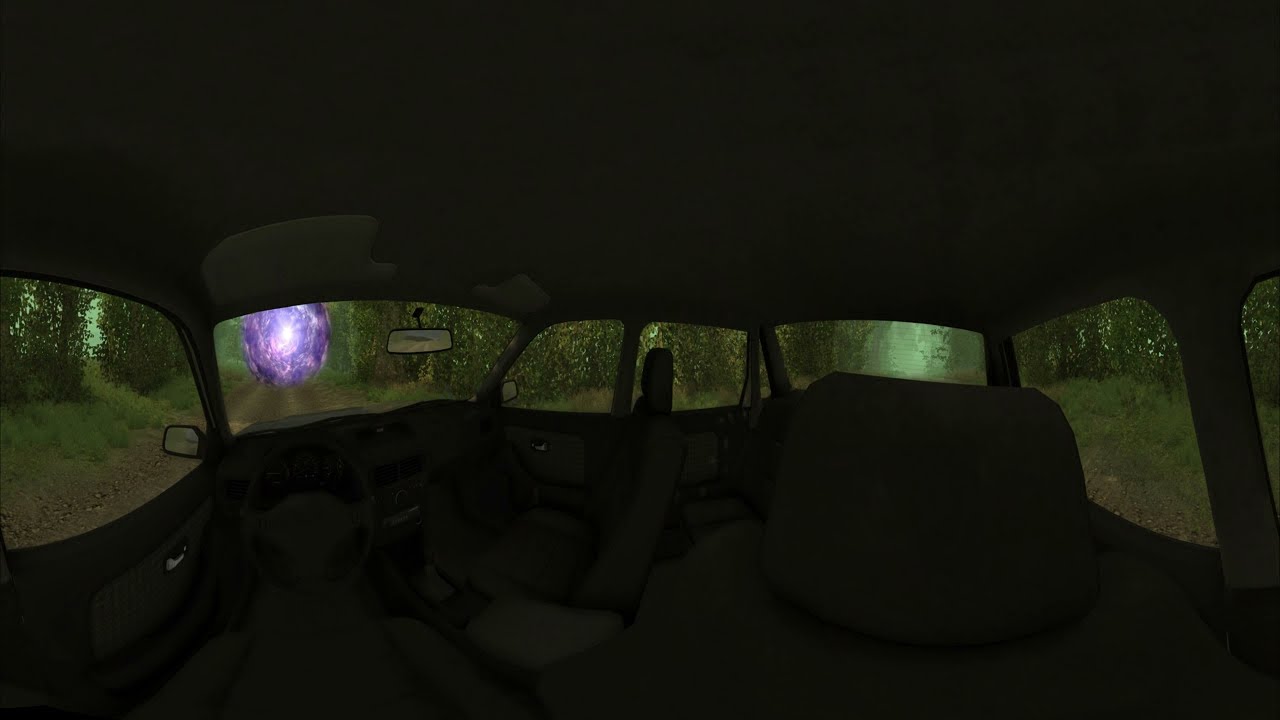The image depicts a dark, eerie scene taken from the back seat of a car. The overall interior of the car is shrouded in darkness, with dark-colored seats and a clearly visible roof interior, including visors and mirrors. The windows, arranged in a U-shape extending from the left to the right, are dotted with what appear to be raindrops, contributing to a blurred, distorted view of the outside. Through these windows, a surreal landscape unfolds; trees and a long dirt road are seen under an unusual, almost supernatural, purple and green glow. This glow permeates the scene, casting an eerie light through the windows and onto the interior, making the image feel otherworldly and hinting at a possibly digital alteration. The image captures an almost jewel-like, circular entity emanating purple light at the end of the road, further enhancing the uncanny atmosphere. The use of a wide-angle or convex lens distorts the perspective slightly, adding to the spooky, dream-like quality of the photograph.